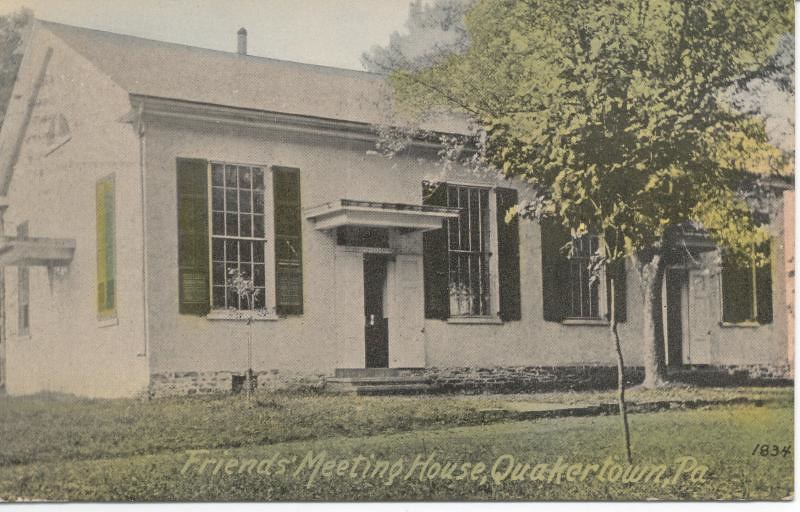This slightly faded and yellowing photograph depicts a historic, white-painted Friends Meeting House in Quaker Town, Pennsylvania, dated 1834. The single-story structure features a modest, traditional design with green shutters adorning each of the four front windows. Each window has 12 rectangular glass panes on both the top and bottom sections. The building's front face also includes two doors, each with a small overhanging roof, mirrored by a similar hangover roof over a side door. A verdant green lawn stretches out in front of the house, accentuated by a couple of trees: one thick and prominent, the other thin and less substantial. The photo displays the name "Friends Meeting House, Quaker Town, Pennsylvania" in yellow script, blending with the photograph's aged hues. In the bottom right corner, "1834" appears in black. The house, possibly serving as a public meeting space, retains additional details such as a potential chimney and a basement or crawlspace indicated by a vent or window at the building’s base.